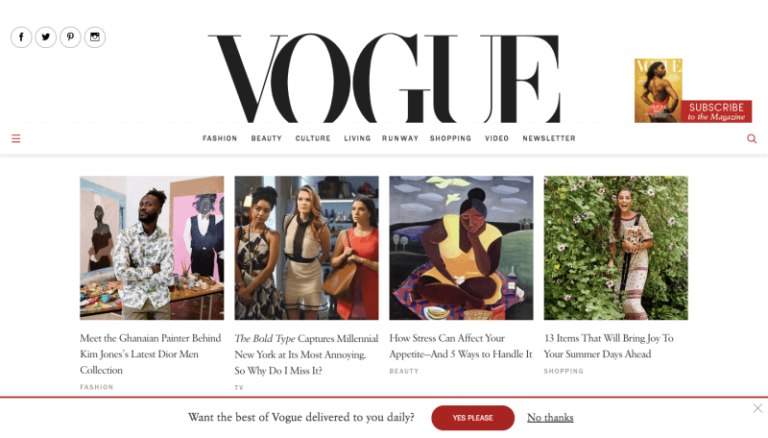Under the "Website" category in the top left corner, there are social media icons for Facebook, Twitter, and Pinterest. Centered just below that section, the word "Vogue" is prominently displayed. Beneath "Vogue," there is a comprehensive menu bar listing various categories: Fashion, Beauty, Culture, Living, Runway, Shopping, Video, and Newsletter.

To the right of the menu bar, there is a small thumbnail image of a Vogue magazine cover. The cover features the back of a person with well-defined muscles, although the image lacks clarity. Accompanying the thumbnail is a call-to-action that reads, "Subscribe to the magazine."

Below this section, four distinct images are displayed horizontally:

1. The first image depicts a woman standing in front of a vibrant wall of flowers. Accompanying this image is the caption: "13 Items That Will Bring Joy to Your Summer Days Ahead" under the "Shopping" category.
 
2. The second image, categorized under "Beauty," discusses mental health with the caption: "How Stress Can Affect Your Appetite and Five Ways to Handle It."

3. The third image shows three women and falls under the "Culture" category. Its caption reads: "The Bold Type Captures Millennial New York at Its Most Annoying, So Why Do I Miss It?"

These captions provide a detailed and organized description of various elements found on the Vogue website's homepage.